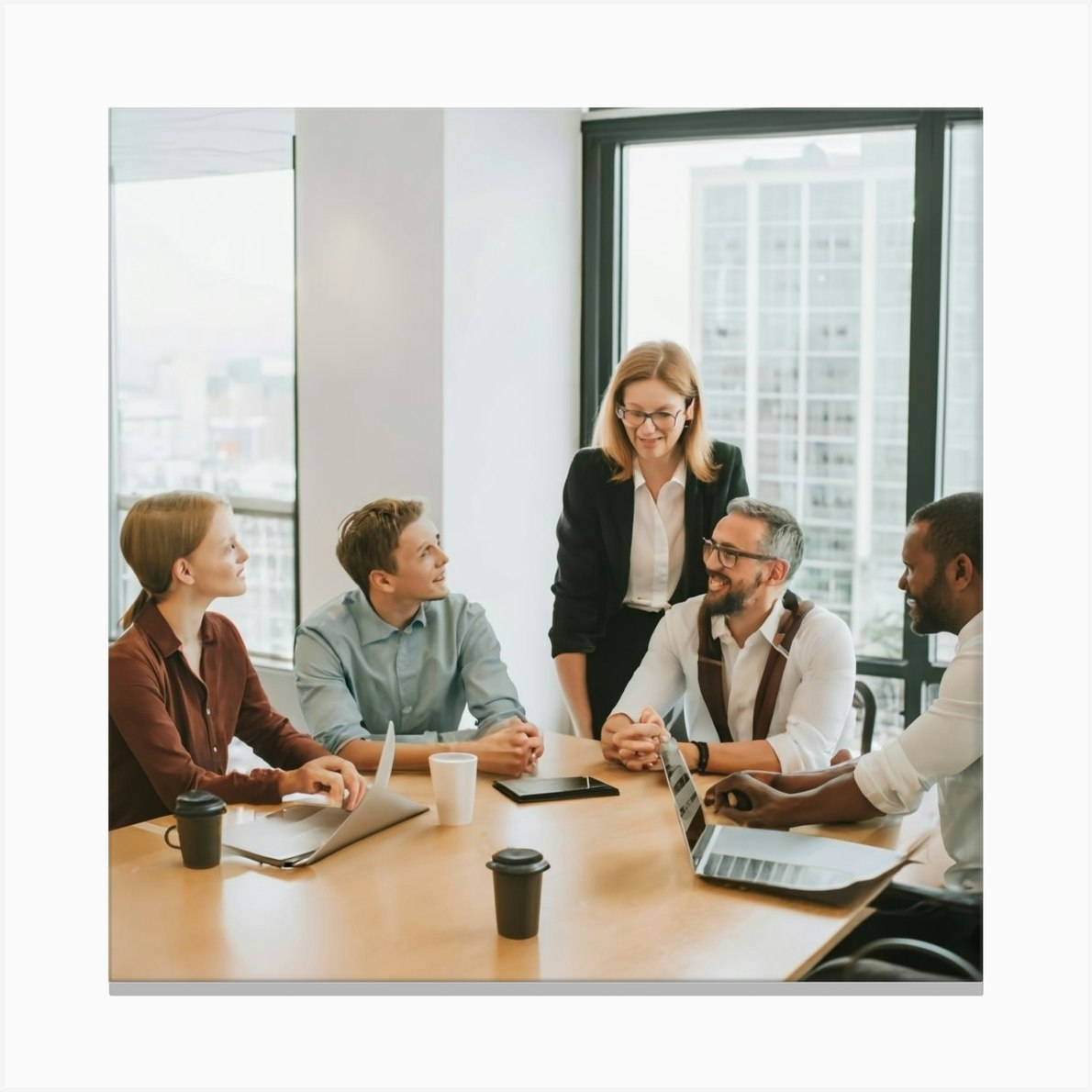In the photo, a professional meeting is in progress inside a sunlit office conference room in a skyscraper. Five people, a diverse mix of ages and genders, are seated around a large tan oak table topped with a couple of oddly-shaped laptops and a tablet. Each participant has a coffee cup, adding to the collaborative atmosphere. To the left, a young woman in a brown shirt gazes to her left while beside her, a young man in a blue shirt shares her direction of look. Standing at the table's end, a middle-aged woman in a white shirt and black blazer oversees another man seated at the table's head, who is looking to his right, dressed in a white shirt with his arms clasped. The far-right chair is occupied by an African-American man who is smiling warmly towards the younger attendees opposite him. Through the large windows behind them, the sunny day outside illuminates part of the meeting area, revealing another skyscraper across the way. The converging smiles and attentive expressions suggest a congenial discussion or brainstorming session.